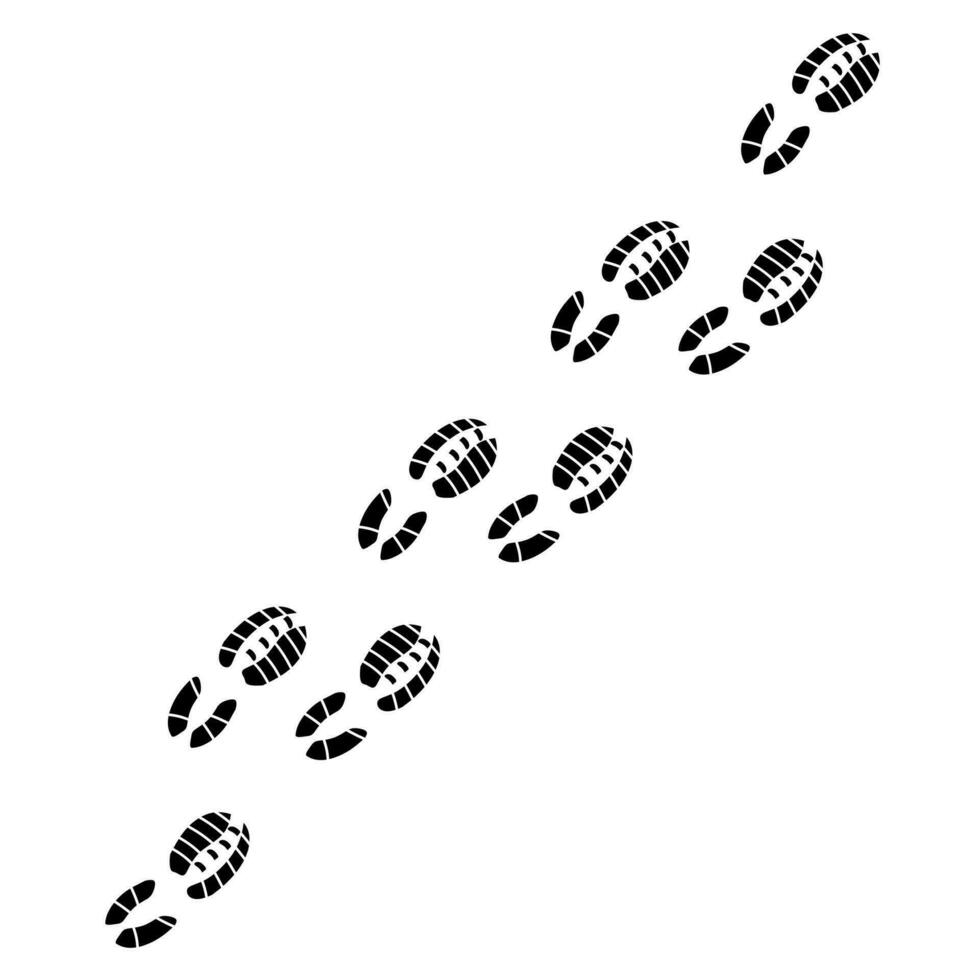The image is a humorous, minimalistic poster set against a white background, featuring a series of black footprints that extend diagonally from the bottom left corner to the top right corner. These footprints, totaling eight in number, are clearly detailed, with the tread patterns characteristic of modern sneakers. Each footprint is outlined in black and segmented by white lines that delineate the sneaker tread, including three black dots in the toe area and two curved black segments at the heel. The footprints include a mix of both right and left prints, distributed in a staggered arrangement. The clever design mimics the appearance of footprints in snow or sand but is presented in stark black on white, emphasizing the humorous and minimalist nature of the poster.